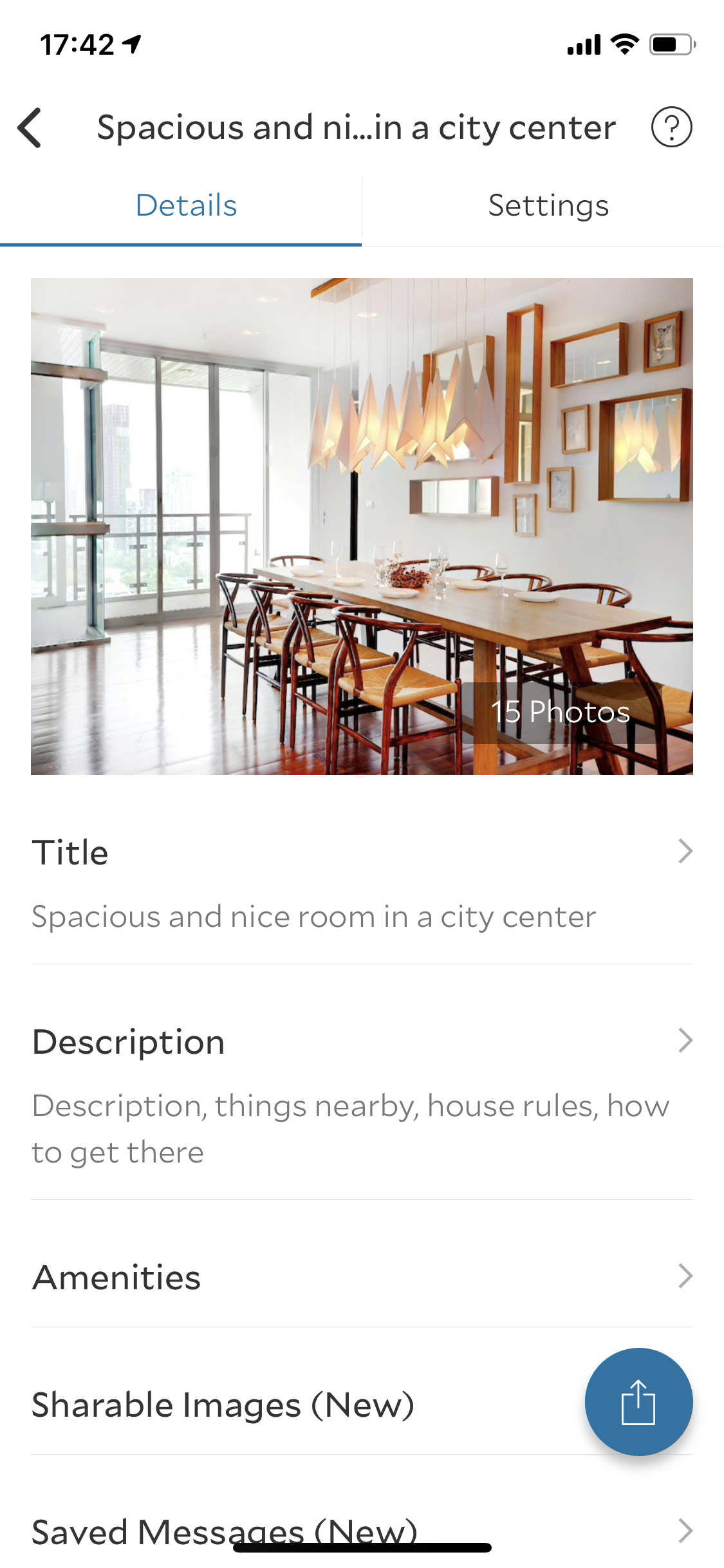Screenshot of a Mobile Interface: At the top-left, the time reads 17:42, with icons including a battery icon on the upper-right. Below this, a header bar displays "Spacious and Nic..in a city center," flanked by a left arrow and a question mark in a circle. The interface is divided into two sections: "Details" (highlighted in blue) and "Settings." A large photograph dominates the screen, showcasing a brightly lit room with several wooden framed mirrors and pictures adorning the walls, a long wooden table, and sunlight streaming through glass windows, casting reflections on the floor. Below the image, various sections with small arrows are listed: 

- Title: Spacious and Nice Room in a City Center
- Description: Including subsections such as "Description," "Things Nearby," "House Rules," and "How to Get There"
- Amenities
- Shareable Images (new) with a blue circle featuring an up-arrow icon next to it
- Saved Messages (new)

A thin black line is centered at the bottom of the screen, indicating the end of the visible content.